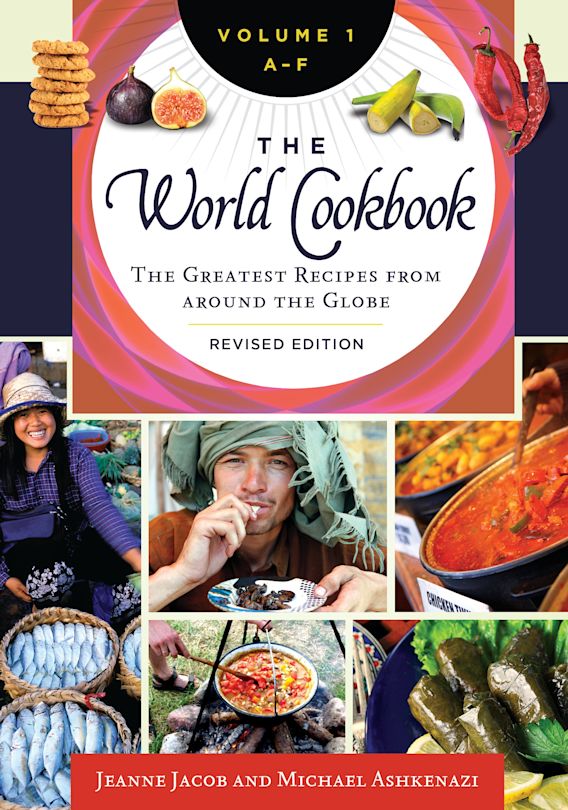The cover of the cookbook is a vibrant and detailed collage that invites exploration of global culinary treasures. Dominated by bold black letters, the title "The World Cookbook," sits within a white circle at the top, followed by the subtitle "The Greatest Recipes from Around the Globe, Revised Edition." Indicating its broader collection, it also specifies "Volume 1, A through F." At the very top, the cover features images of colorful fruits like bananas, chilies, and cookies, hinting at the diverse ingredients you will encounter inside. Below, a montage of five photographs showcases people deeply engaged with food from around the world. A woman beams next to baskets teeming with medium-sized fish, while an ethnic man savors a regional dish, adorned with a green head covering and a brown shirt. Another image displays a person stirring an Italian dish, exuding the warmth of home cooking. A tomato-based salsa or similar dish shares the spotlight, along with an elegantly plated vegan appetizer. Nestled in the bottom right corner, names of the authors, Jean Jacob and Michael Ashkenazi, lend authority to this compelling culinary compendium.